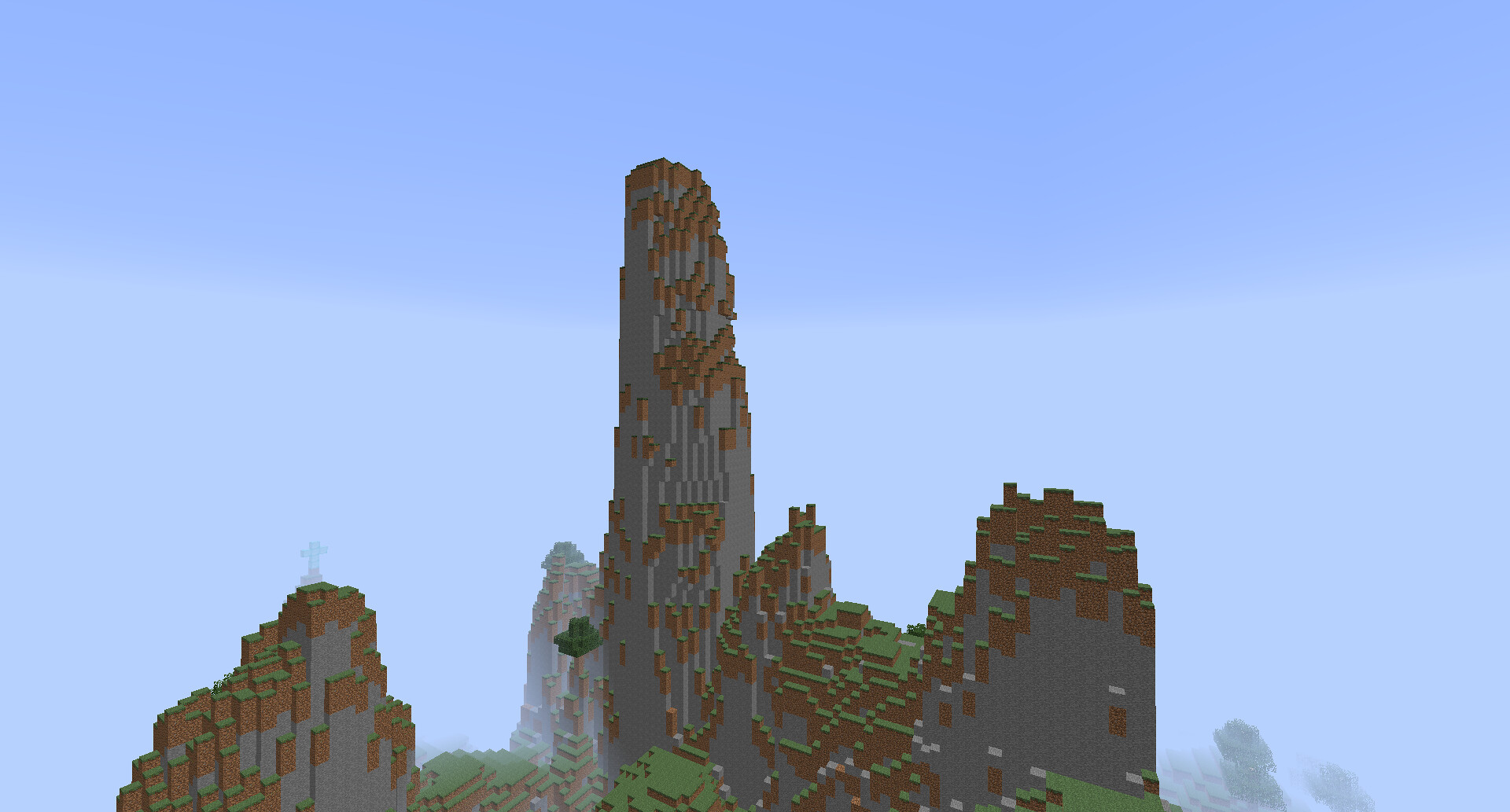A digitally generated image resembling a pixelated or Lego-constructed landscape. An expansive blue sky occupies approximately 75% of the background, with a gradient transitioning from a deep blue at the top to a lighter blue toward the middle and bottom. Dominating the foreground is an intricate, Lego-like mountain composed of thin, gray Lego bricks. This towering structure features brown and green accents scattered across its surface, mimicking rock formations, vegetation, or architectural elements. The mountain rises majestically in the center, reaching its highest peak like a spire. On the bottom left, a smaller rock or mountain formation provides additional depth. The structure extends to the right with various sub-peaks and troughs, suggesting the outline of a castle or a series of connected buildings. The overall composition creates an intriguing blend of natural and constructed elements, rendered in a simplistic yet detailed pixelated style.